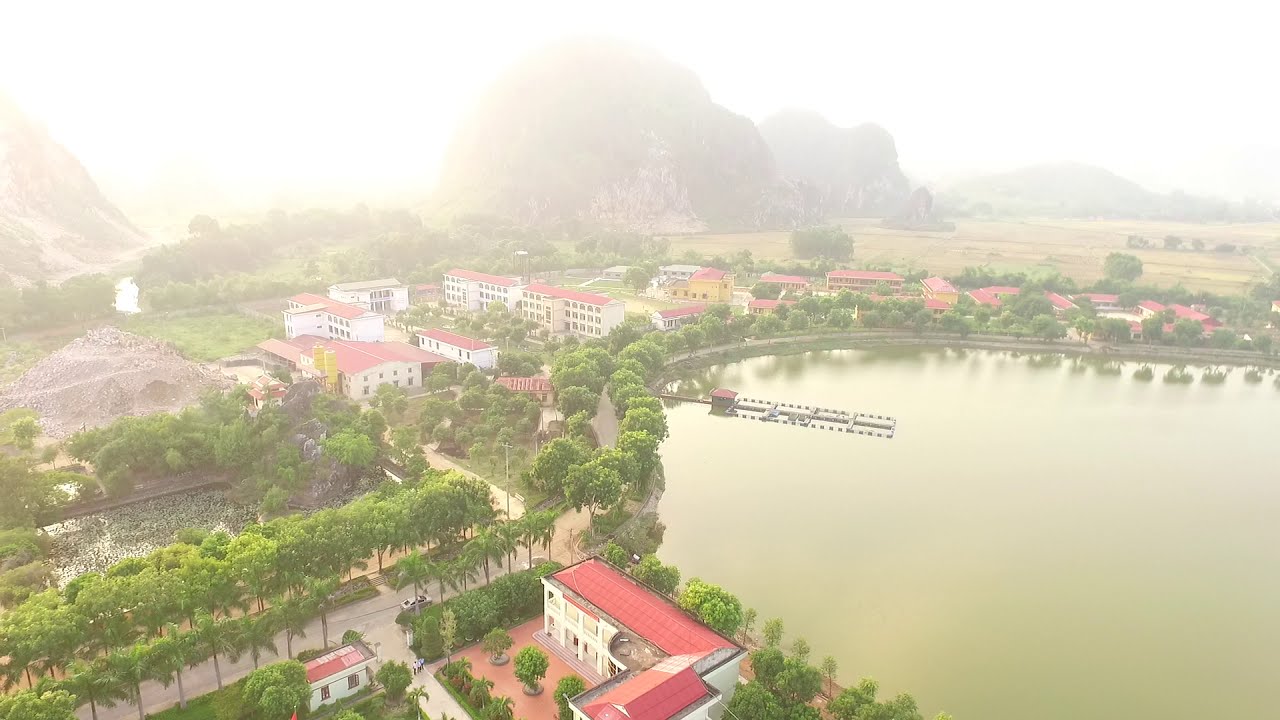From a high-angle perspective, the image captures a serene East Asian town enveloped in a hazy, dream-like glow, possibly due to dust or fog in the air. The scene centers around a calm, brown lake occupying the bottom right of the image, bordered by a marina or dock with no visible activity. Surrounding the lake, multi-story white buildings with terracotta red roofs, reminiscent of structures from the 1940s or 50s, are interconnected by roads lined with a mix of palm and green trees. These buildings, which could be hotels or various facilities, cluster densely in the central and bottom areas, forming a cohesive community. In the background, the imagery shifts to softer tones with diffused light outlining rocky, round peaks that jut from the ground, adding an inviting, almost ethereal quality to the landscape. The top of the image remains blurry, with a bright white sky, enhancing the overall softness and tranquility of the scene. To the left, tall trees and light brown fields extend upward, while a car is faintly visible on a road in the bottom left, emphasizing the calm and stillness of this picturesque town.